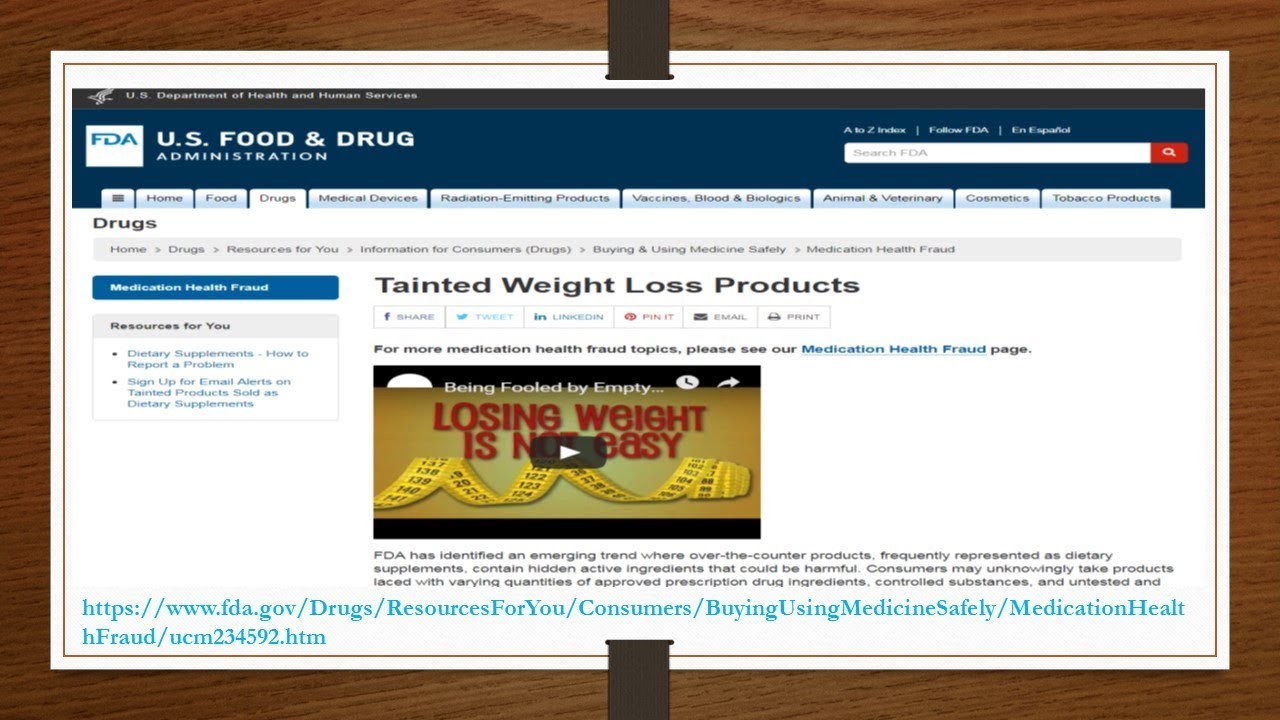A meticulously edited screenshot of the US Food and Drug Administration (FDA) website framed with a wooden border. Prominently featured at the top left is the FDA logo, while the search bar, accented with a red magnifying glass icon, resides on the top right. The top banner is a bold navy blue ribbon, hosting various navigational tabs. From left to right, these tabs display icons and labels: a male symbol, Home, Food, Drugs (the active tab), Medical Devices, Radiation-Emitting Products, Vaccines, Blood and Biologics, Animal and Veterinary, Cosmetics, and Tobacco Products.

The active 'Drugs' tab leads to an article titled "Tainted Weight Loss Products," seen beneath a set of navigational breadcrumbs. Below the article title are sharing icons for Facebook, Twitter, LinkedIn, Pinterest, email, and print. The article features text explaining the issue and includes an embedded YouTube video with a partially visible title "Losing Weight is Not Easy" and a cut-off title "being fooled by empty...". Additional informative text follows, accompanied by a sidebar on the left containing further resource links.